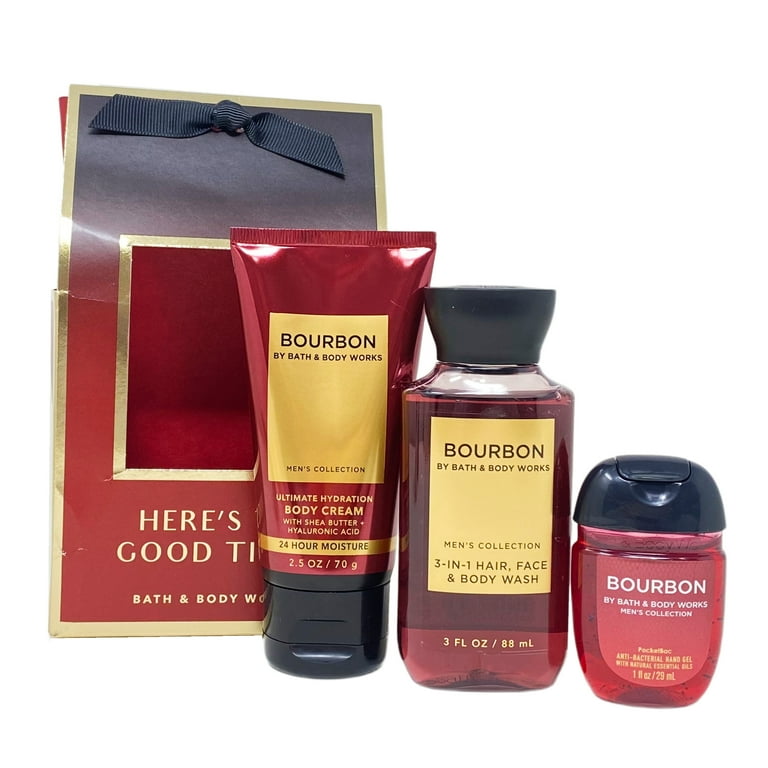This image showcases a curated set of Bath & Body Works men's beauty products, prominently featuring the Bourbon collection. The ensemble includes four distinct items arranged from tallest to shortest, left to right. The largest item is an ultimate hydration body cream enriched with shea butter and hyaluronic acid, promising 24-hour moisture. Next, there's a 3-in-1 hair, face, and body wash, contained in a 3 fluid ounces bottle. The smallest item seems to be an antibacterial hand gel, estimated at around 1 fluid ounce. Each product showcases a visually appealing packaging in hues of red, black, and gold, with the collection title "Bourbon" clearly displayed. Additionally, there is a burgundy and black gift bag adorned with a black bow and the phrase "here's to good times" in gold lettering, adding an extra touch of luxury. All products appear to be offered as part of a coordinated men's care set, ideal for gifting or personal use.